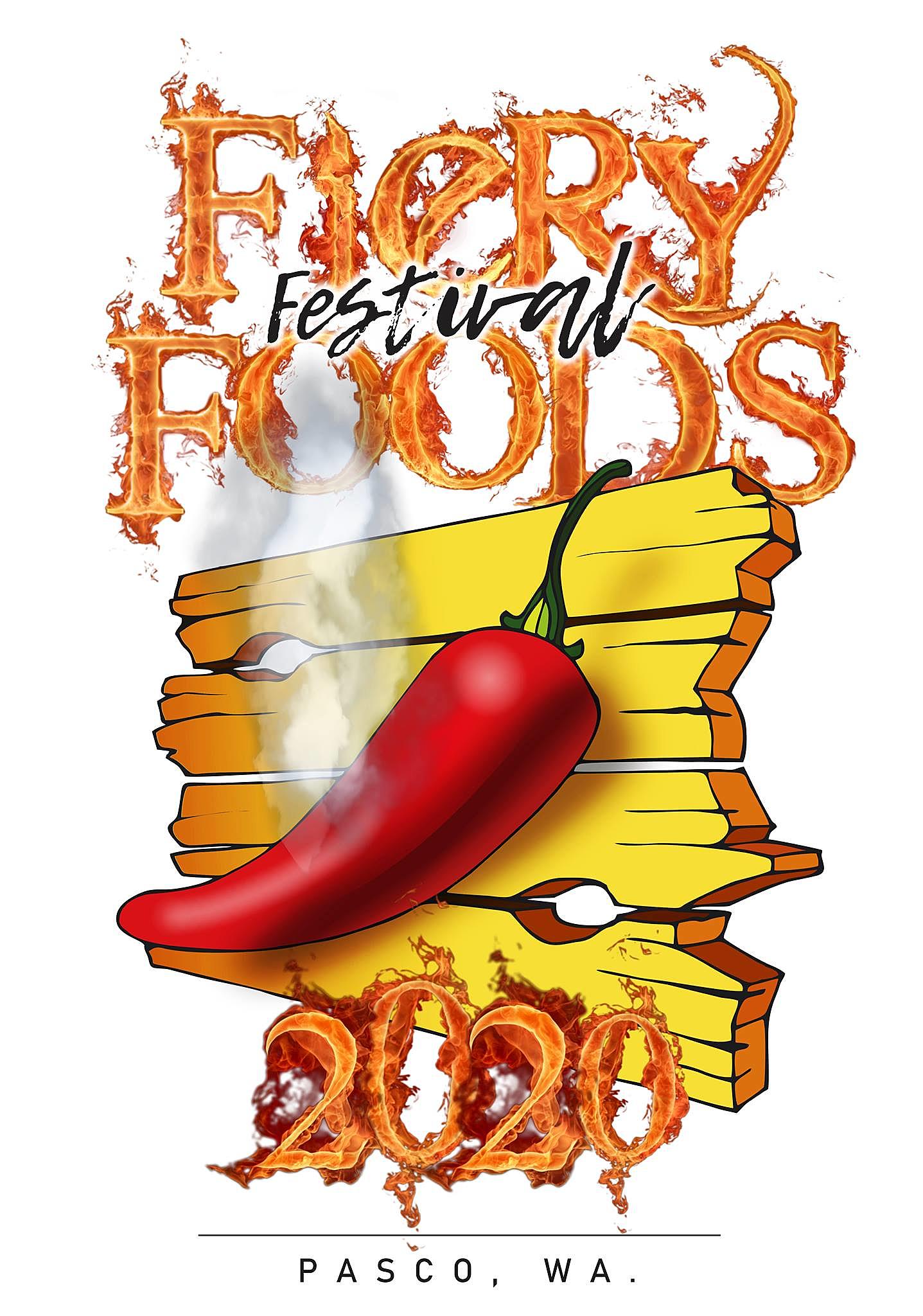This digital rendering showcases the vibrant logo of the "Fiery Foods Festival 2020" held in Pasco, Washington. The main elements of the logo are the words "Fiery" and "Foods," both rendered in a dynamic, sans-serif font designed to appear as if they are engulfed in flames, giving it a fantastical and intense visual appeal. Between "Fiery" and "Foods," the word "Festival" is elegantly scripted in a handwritten font, adding a touch of whimsy and personalization. 

Beneath the main text, "2020" is repeated twice in the same flaming font, reinforcing the year of the event. Below it, "Pasco, WA" is clearly printed in a clean, sans-serif typeface to provide location clarity. Central to the composition is a large, distressed wooden plank split into several pieces, adding a rustic and rugged feel to the overall design. Dominating the foreground is an oversized, bright red chili pepper with a vivid green stem, symbolizing the spicy theme of the festival. The entire image, as a digital rendering, combines fiery elements with bold text to create an eye-catching and thematic representation of the event.